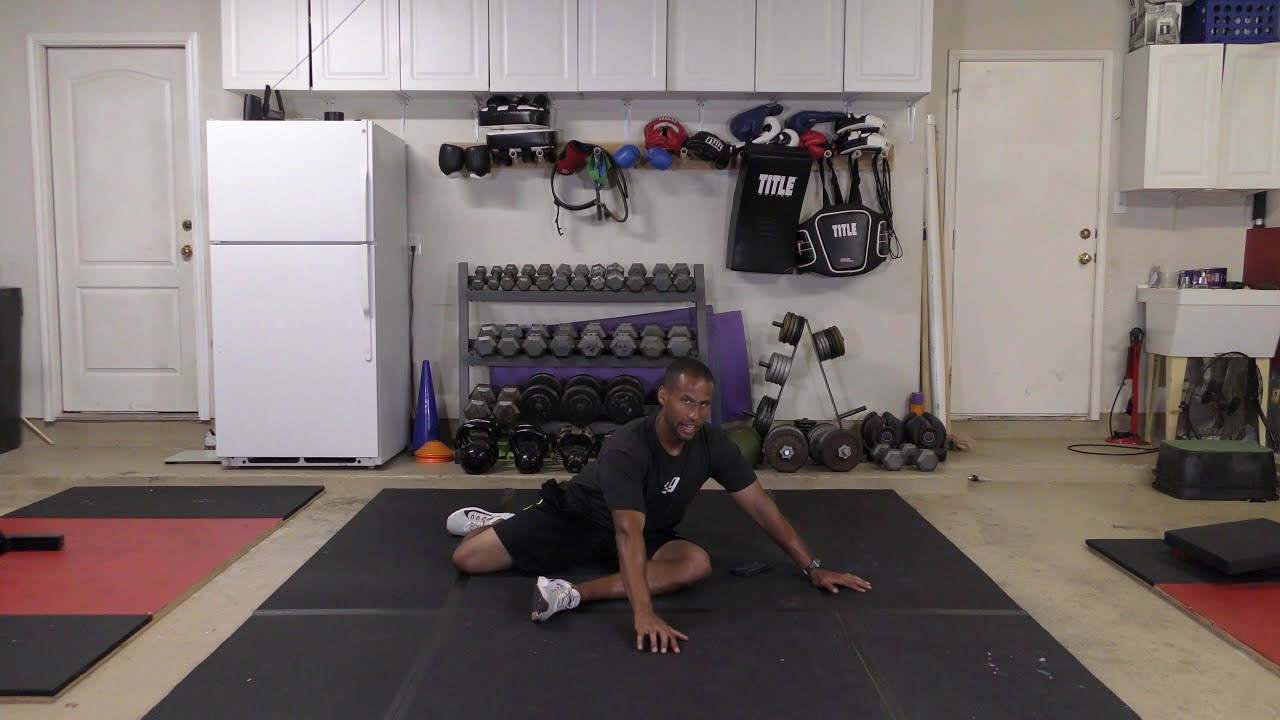In this detailed photograph, we see a black man positioned on a black exercise mat with darker black strips dividing sections. The concrete floor and surroundings suggest that he is in a garage, which has been repurposed into a makeshift gym. The man has short black hair and is attired in black athletic shorts, a dark gray t-shirt featuring an indistinct white emblem at the center, and white sneakers. He wears a watch on his left wrist and is situated on his hip, with one leg under him and the other stretched out in front.

His fingers are splayed on the mat behind him as he seems to be engaging in a stretching routine while looking towards the camera, possibly speaking. Directly behind him, a rack filled with various dumbbells – gray and black – is organized, with lighter weights arranged higher up. Surrounding this area, the back wall is predominantly white with some gray patches. To the left of the weights is a white refrigerator topped with closed white cabinets. Additionally, white doors frame both ends of the background, adding symmetry to the scene. This vividly captures a man in the middle of his workout regimen in a well-organized home gym setup.